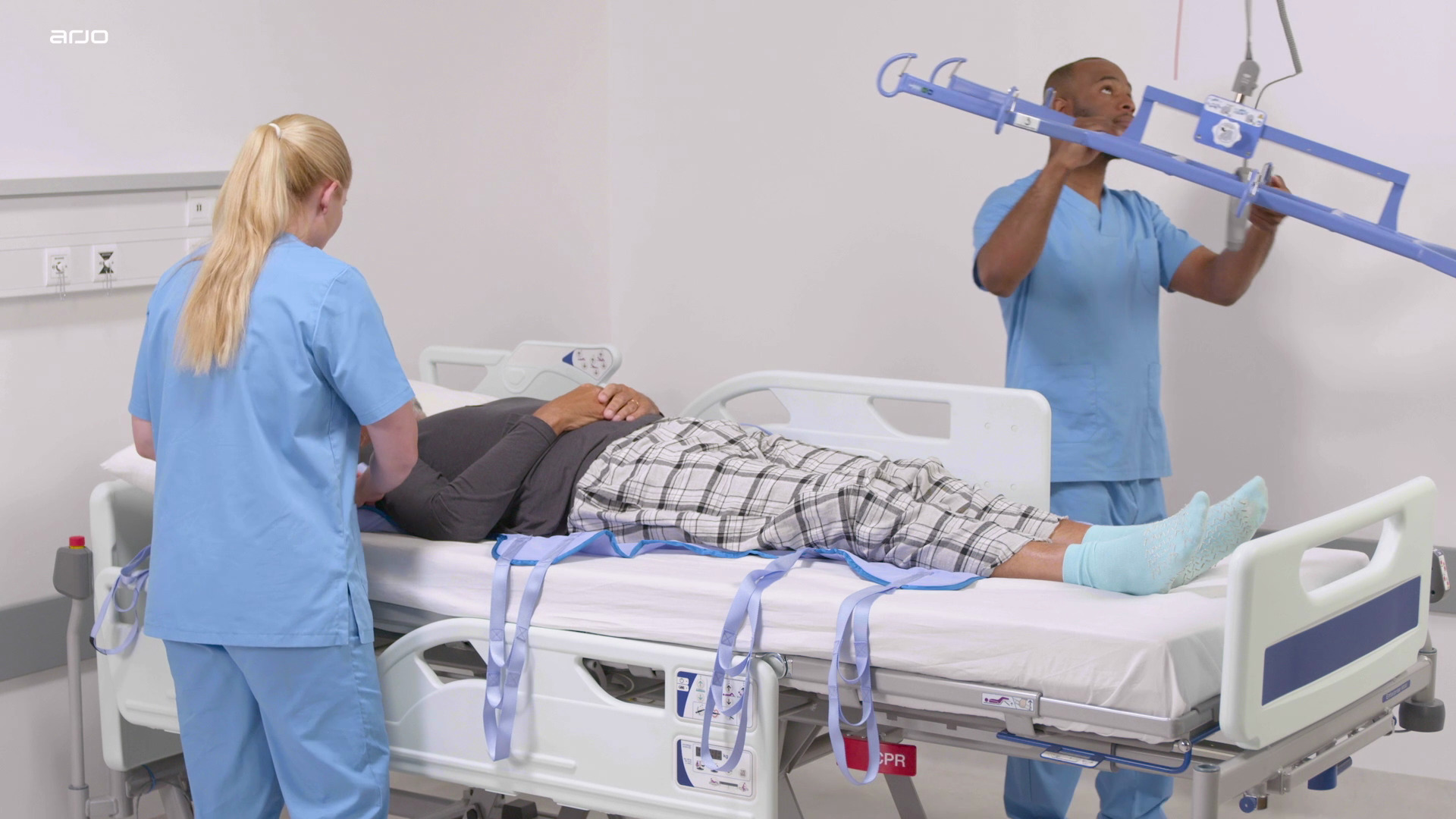The image depicts a stark hospital room with white walls and minimal furnishings. At the center of the image, a patient is lying on a hospital bed, wearing white and gray plaid pajama pants, a long-sleeve gray top, and very light teal or white socks. Underneath the patient is a pad with three sets of strings or ties visible, associated with a Hoyer lift—an assistive device for patients who cannot move independently. 

To the left, at the head of the bed, stands a female nurse with blonde hair. Her back faces the camera, obstructing a view of her face, and she is dressed in light blue scrubs. On the right side of the image, a male nurse with dark skin, who is balding, is setting up the Hoyer lift. His scrubs are slightly darker compared to the female nurse’s. 

Both nurses are focused on their tasks; the female nurse appears to be overseeing the patient, while the male nurse is in the process of adjusting the equipment. In the upper left-hand corner of the image, the barely discernible letters “ADO” are faintly imprinted, blending into the light background. The overall scene is clinical and utilitarian, emphasizing the essential care being provided to the patient.